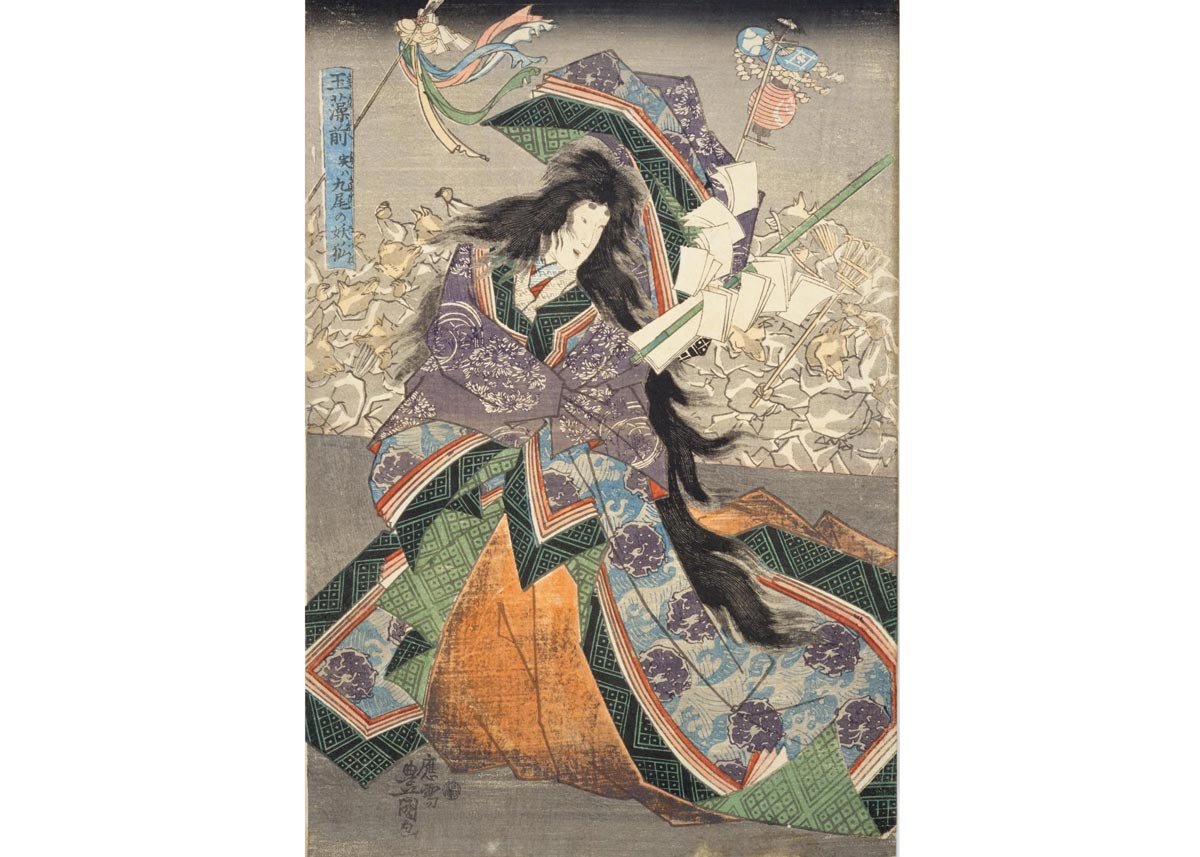The image depicts a sophisticated piece of traditional Japanese art, characterized by its detailed and intricate painting style. Dominating the center of the scene is a woman, or perhaps a nine-tailed fox in disguise, dressed in an elaborate traditional kimono. The kimono is adorned with a multitude of colors and patterns, including blue waves, purple flowers, a green hem, dark orange skirt, and a purple shawl. A yellow fabric and cherry blossom patterns accentuate the garment's complexity. She is holding a paper lantern and a bamboo stick that extends towards the right side of the image.

On the left-hand side of the artwork, there is a vertical blue banner featuring black calligraphy, which serves as a caption or perhaps the artist's signature. The background of the image is a grey expanse at the top with a tumultuous scene unfolding below. The scene appears to depict a battle, with various figures—be they humans or anthropomorphic foxes—engaged in combat, wielding different objects. The setting and characters suggest a rich narrative steeped in Japanese mythology and artistic tradition.